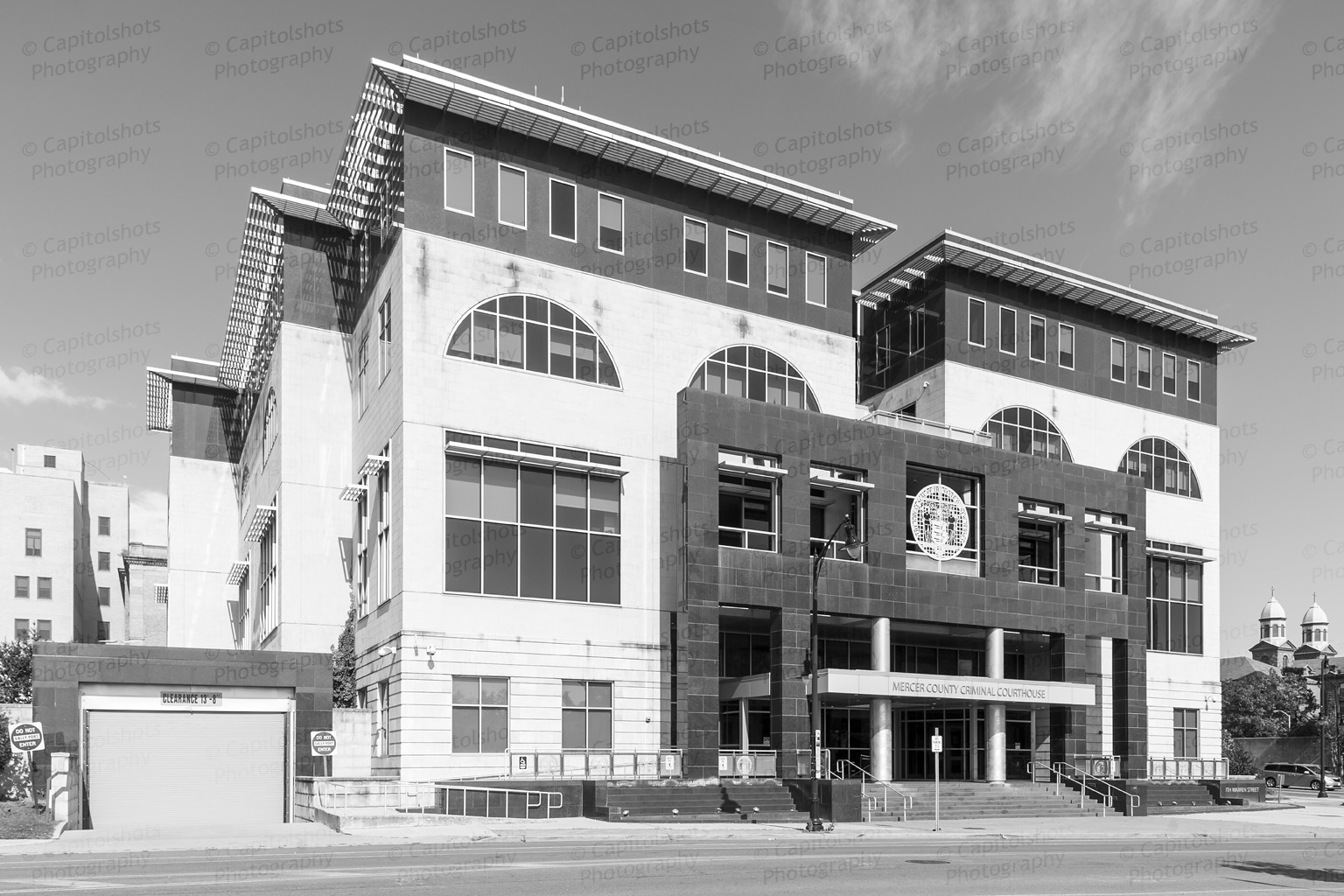This black-and-white photograph captures the Mercer County Criminal Courthouse, identifiable by the text inscribed on the gray steel beams at the entrance of the building. The image, in a wide vertical rectangular format, prominently features the courthouse slightly offset to the right with a visible one-flight staircase leading up to the open lobby. The building showcases a brick facade and appears to be three stories in height, with additional structures within that create a gap at the top, giving the illusion of a less cohesive structure. The two vertical rectangular columns of the building, joined by a walkway, are white up to the top floor before transitioning to gray, capped with flat roofs projecting over the edges. A paved road is visible at the bottom of the image, and to the left, a garage can be seen. The background reveals the tops of other concrete buildings under a gray sky. Watermarked with "Capital Shop Photography," this detailed composition highlights the courthouse's architectural elements amidst its urban surroundings.